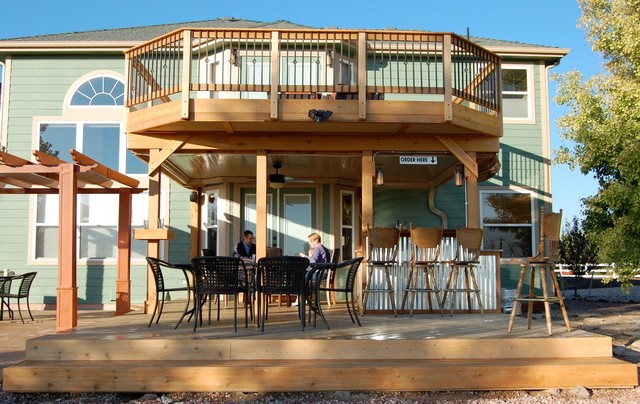The image depicts the outdoor area of a two-story restaurant that closely resembles a traditional sage green home, complete with distinctive, large windows, including a semi-circular one with split panes. A spacious wooden balcony is positioned above a wooden deck, both constructed from unpainted wood. The scene is bathed in daytime sunlight under a clear medium blue sky, with a tall tree featuring thick green foliage standing on the right. Black metal furniture populates the deck, including a table and six chairs. Closer to the house, two individuals are seated at another table set, engaged in conversation. To the right, there is a small mini bar marked by a sign that reads "order here," with three tall chairs in front of it. A lighter wood trellis, currently flowerless, adds charm next to the deck. The overall setting exudes a cozy, home-like atmosphere with a hint of vintage allure, further enhanced by a white picket fence and a wooden canopy.